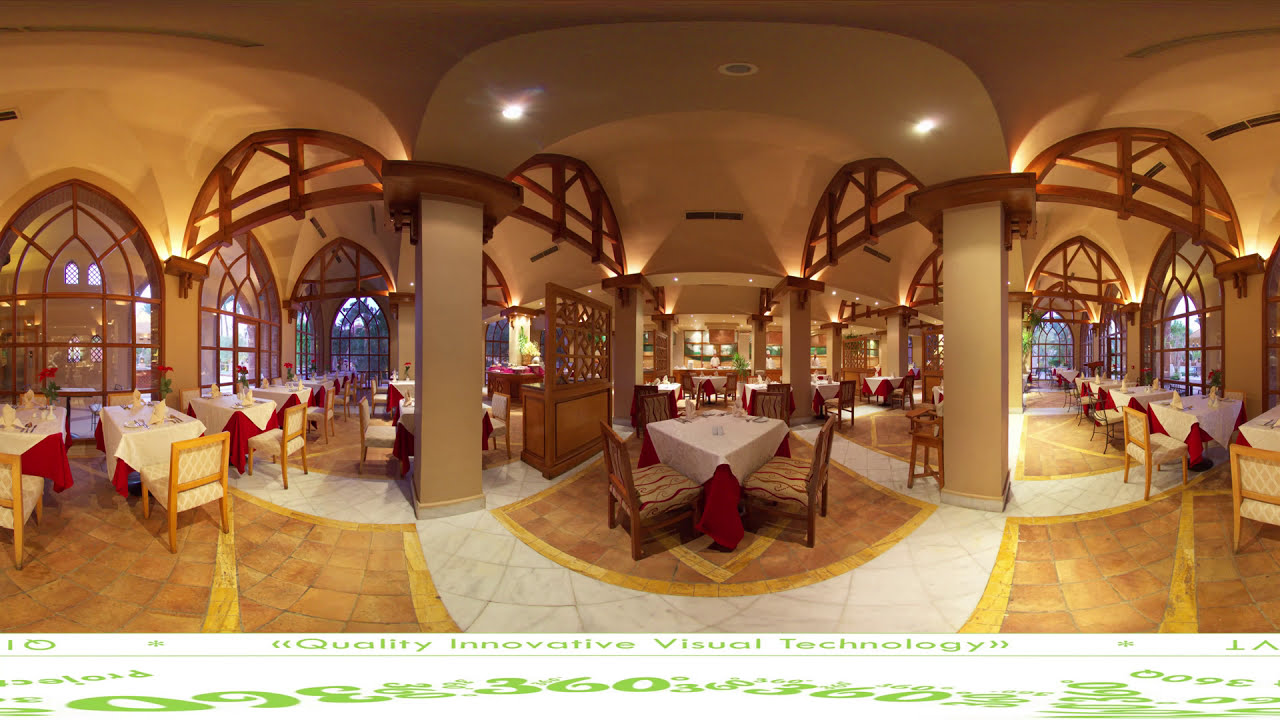The image showcases a 360-degree panoramic view of a grand restaurant interior, slightly warped due to the panorama effect. The spacious room is bathed in beige tones and is divided into three distinct sections. The restaurant features a multicolored, predominantly tan-tiled floor, accented with white tiles and gold edges along the periphery.

Each section of the restaurant is furnished with square tables dressed in dual-layered tablecloths: a red cloth underneath a white one. The tables are organized in rows, with two-person tables aligned on the right and left sides, and four-person tables placed centrally. Every table is elegantly set with upright napkins and flower centerpieces. The chairs differ in color, with the central tables adorned with darker brown seating, while the side tables feature lighter, brighter wood chairs.

Two rectangular columns, supported by dark wood beams, stand prominently in the middle of the space. Tall, arching pillars with wood accents enhance the room's structural elegance. The walls and ceilings are designed with multiple arch-shaped windows with brown frames, allowing natural light to seep through. Additionally, scattered white lights add to the ambient lighting. 

At the bottom of the photo, a white strip highlights the phrase "quality innovative visual technology," repeated with the figures "360" in various orientations. The overall setting suggests a sophisticated dining environment characterized by meticulous attention to detail and a harmonious blend of colors and textures.